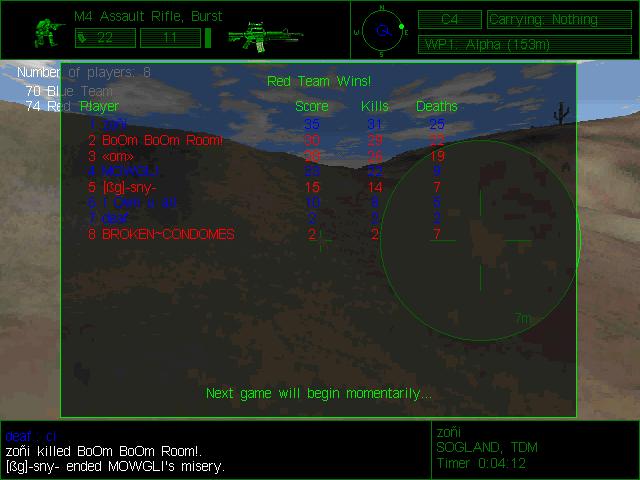In the ongoing video game, the background scene features expansive desert sand dunes under a clear blue sky, giving a stark but scenic backdrop. Dominating the central focus, the game itself is confined within a black bordered square. At the top of this section, prominent red lettering proudly announces, "Red Team Wins." Below, a notification assures players that the "Next game will begin momentarily."

The screen meticulously lists different categories for scoring, kills, and deaths, providing a comprehensive breakdown of in-game performance. Across the lower portion of the screen, a black banner with bold white text states, "Zoni killed boom boom room!" adding an exclamatory flair to the victory announcement. The immersive visuals and detailed notifications combine to create a vivid portrayal of the culmination of an intense gaming session.